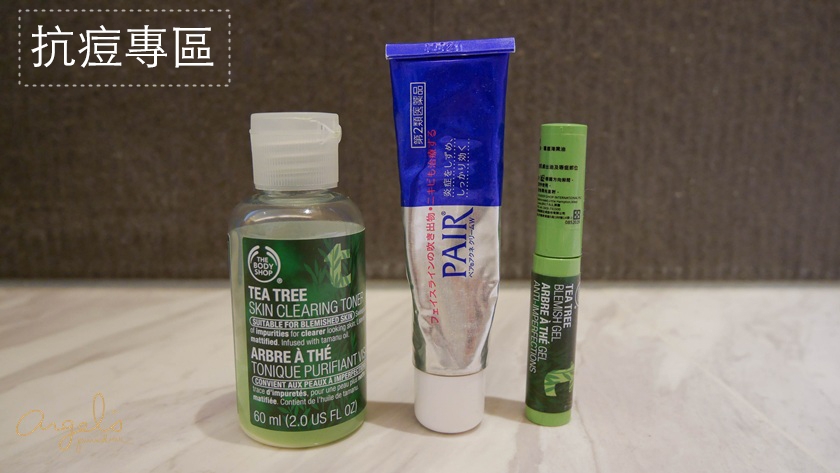This horizontally oriented image displays three distinct products on a pristine, white marble-like surface. On the left, there is a Tea Tree Skin Clearing Toner, contained in a small plastic bottle filled with a light green liquid. The bottle is topped with a white plastic cap that lifts to reveal an applicator hole for dispensing the toner. 

In the center stands a tube with a white cap at its base. The upper half of this tube features a blue background, while the bottom half is a solid, silvery color. Prominently displayed on the front is the blue word "Pear," accompanied by additional red and blue text as well as script in an oriental language.

To the right is a narrow, cylindrical container labeled "Tea Tree Blend Gel." The label is predominantly black with gray and white lettering, and it boasts a green cap that remains encased in its original clear plastic wrapping, complete with small black text. 

In the upper left corner of the photograph, a white box displays a series of disjointed lines forming Chinese characters. The backdrop of the image is a brown, fabric-like wall, offering a neutral and textured contrast to the sleek surfaces of the products.